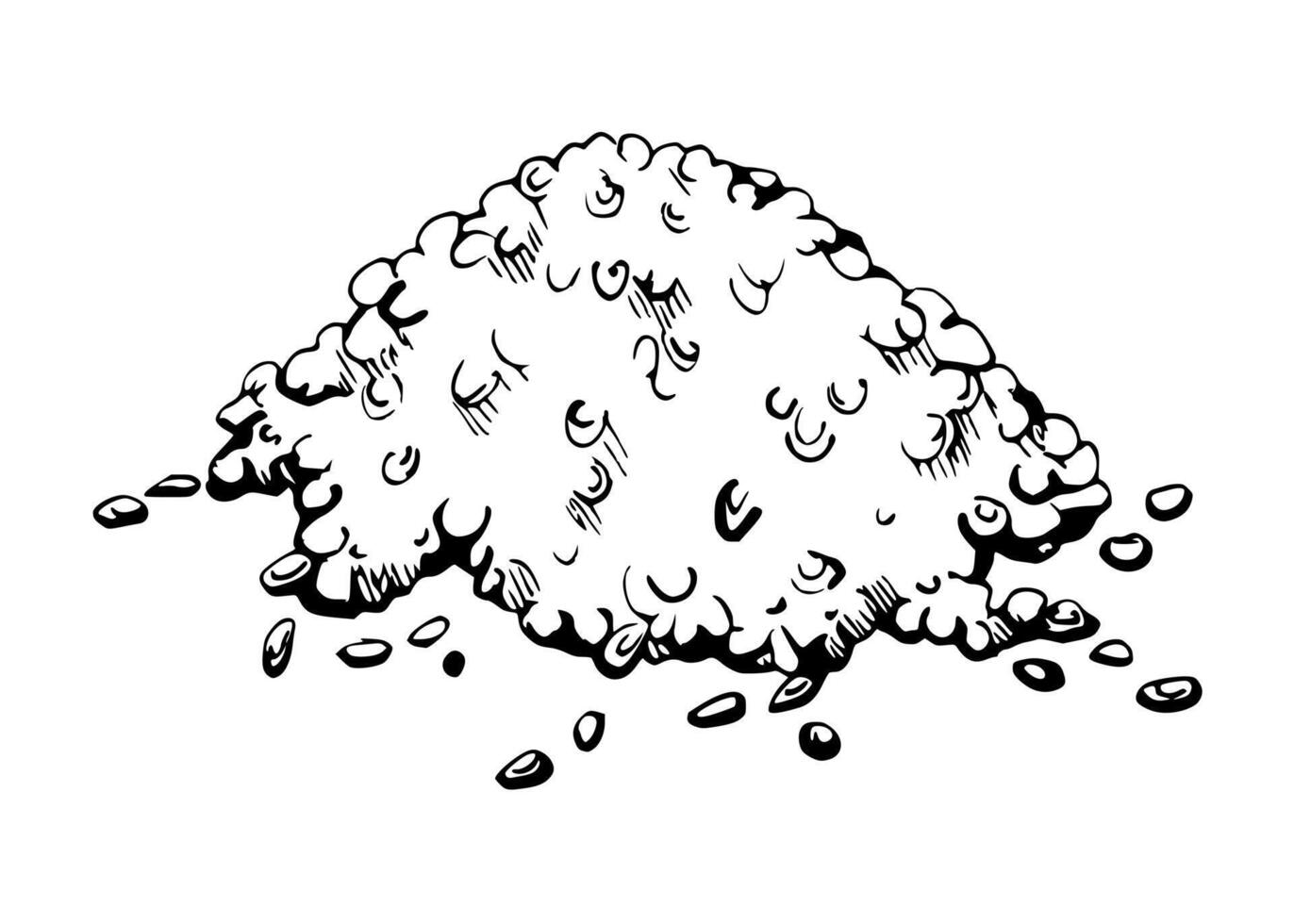This is a black and white, computer-generated drawing that depicts a large, central pile of small, oval-shaped objects that resemble beans, seeds, or possibly pebbles. The objects, outlined in thick black lines, vary in size and shape, with some appearing more rounded or circular. The pile has a jagged, uneven base, emphasized by a thick black line to imitate shadow. At various points within the pile, some objects feature black lines or hooks, suggesting extraneous details or texture. Scattered around the base are several individual objects that have separated from the main heap. The background of the image is entirely white, providing stark contrast to the detailed, line-drawn objects. The style of the drawing is somewhat simplistic, akin to a comic or cartoon, with minimal shading and a focus primarily on the outlines of the shapes.